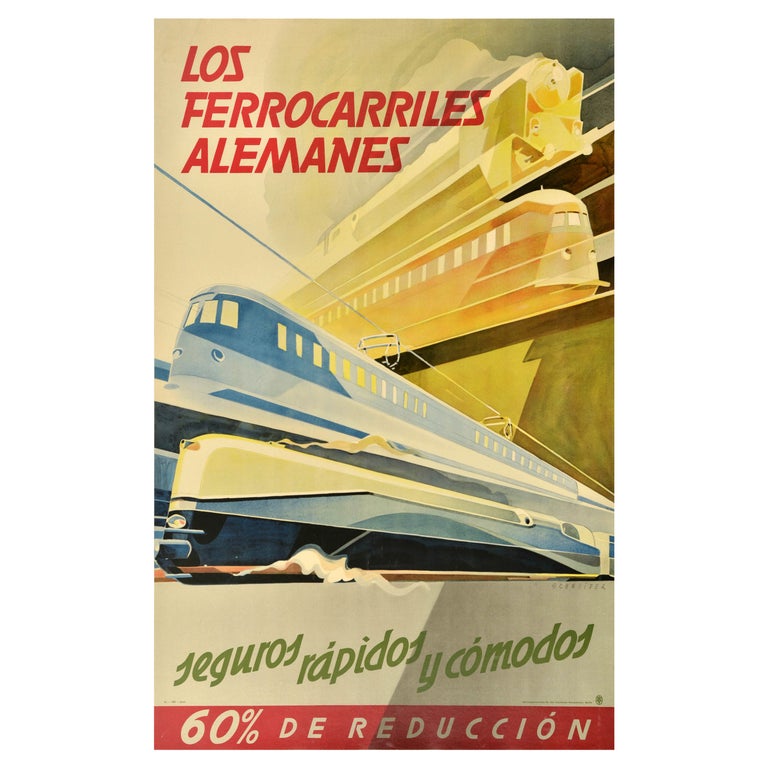This advertising image for "Los Ferrocarriles Alemanes," which translates to "The German Railways," features a vintage-style illustration, emphasized by its yellowed coloring. The artwork consists of watercolor-painted trains, arranged in two rows. The top row displays two yellow and orange-hued trains heading towards the right, with one utilizing coal for power. The bottom row shows two predominantly blue trains traveling to the left; one is an electric train connected to overhead catenary wires, while the other appears to emit steam from underneath. The image includes Spanish text in red, green, and beige, with the top left corner reading "Los Ferrocarriles Alemanes," and the middle of the image stating "Seguros, Rápidos y Cómodos," meaning "Safe, Fast, and Comfortable." At the very bottom, a red banner announces a "60% de reducción," indicating a significant discount.